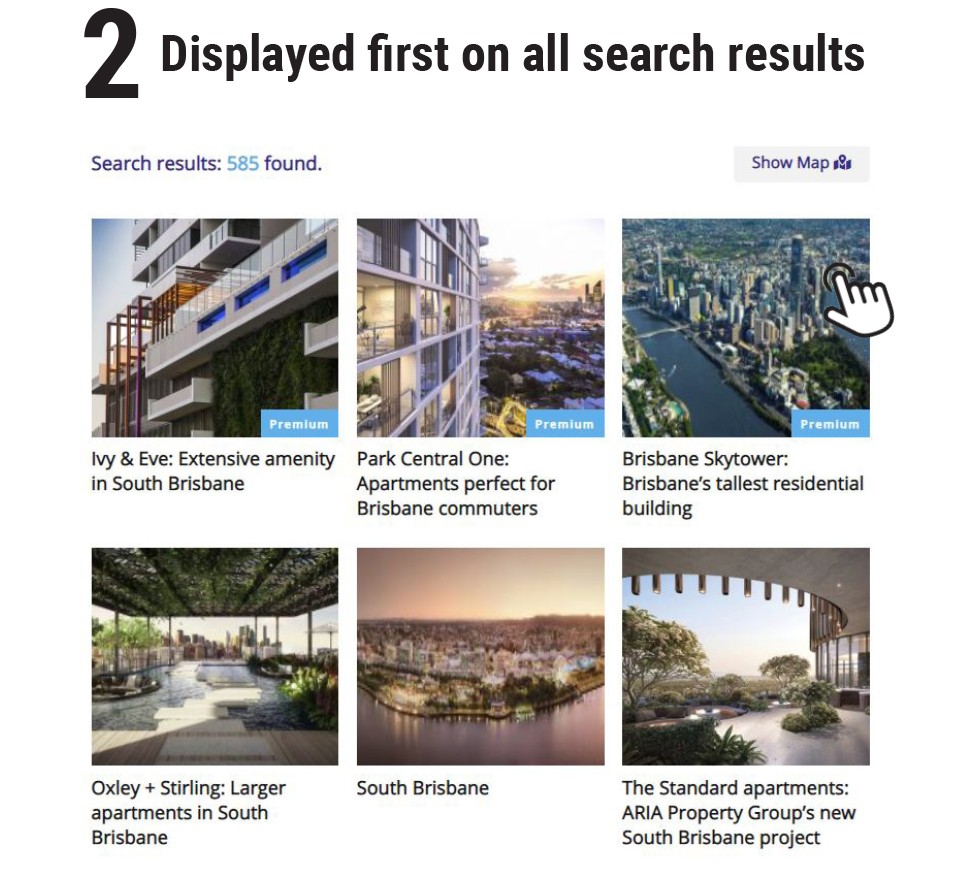The image is a screenshot of a search engine results page, featuring a variety of listings in large, bold black font. At the top of the page, the text "2." is prominently displayed in a big, bold font. Underneath it, in a smaller blue font, the phrase "Displayed first on all search results" is visible. Additionally, the number "585" is written in a lighter blue font, indicating the total number of search results found.

In the upper right corner of the image, the option "Show maps" is available. The cursor, depicted as a white hand, is also visible on the screen. 

The first search result showcases "Ivy and Eve", described as an extensive amenity in South Brisbane. This premium location features a modern building with exterior plants climbing its sides. A pool is visible on one of the upper floors along with glass cutouts adorning the building.

The second listing presents "Park Central 1", noted for being an ideal apartment complex for Brisbane commuters. The image accompanying this listing displays a high-rise luxury apartment complex offering a breathtaking view of the city.

Finally, the third search result features "Brisbane Sky Tower", identified as Brisbane's tallest residential building. The accompanying aerial shot captures a panoramic view of the city alongside a notable waterway.